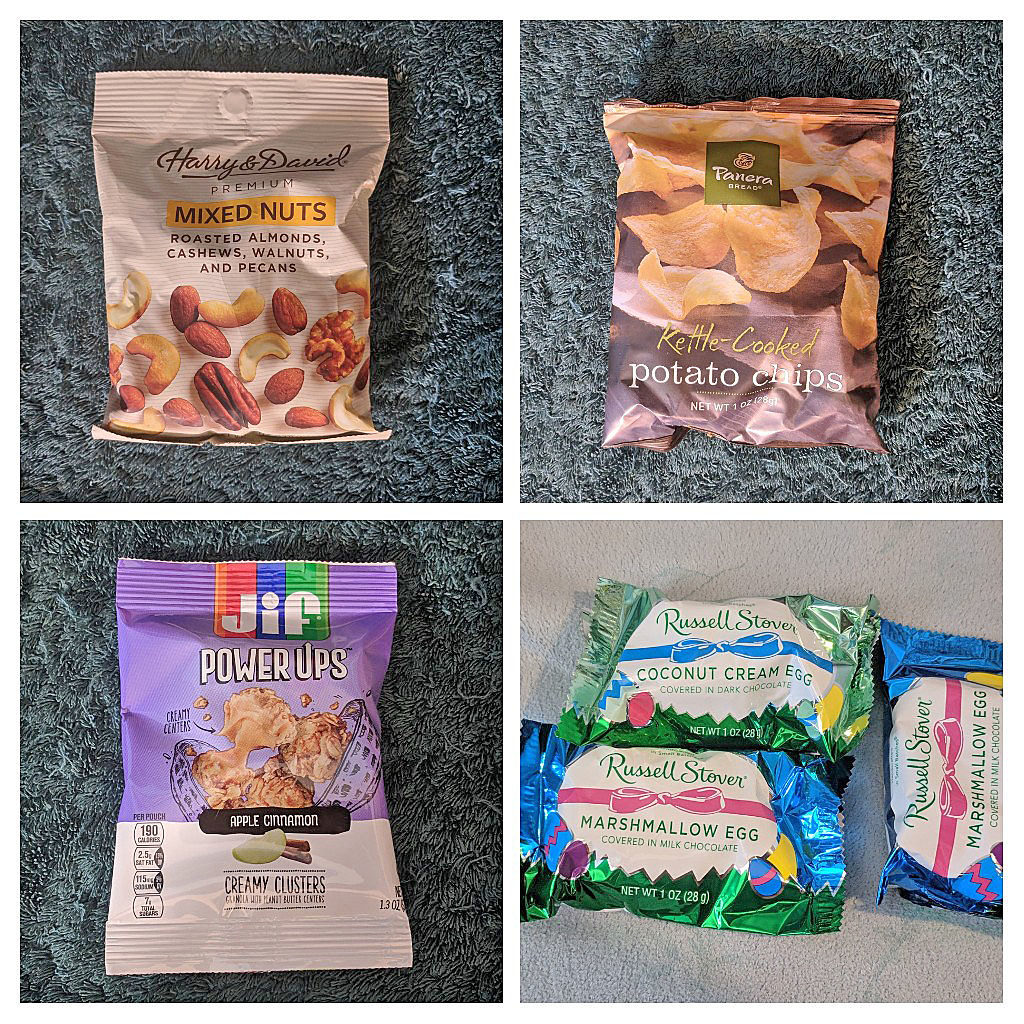The image showcases a neatly arranged grid of four equally spaced photos, each depicting a different snack package against a consistent bluish-gray background, except for the bottom right photo with a white background. 

In the top left corner is a tan-colored bag labeled "Harry and David Premium Mixed Nuts," featuring illustrations of roasted almonds, cashews, walnuts, and pecans. Directly to its right, there's a Panera Bread branded bag of kettle-cooked potato chips, accompanied by an image of the crisps themselves. 

On the bottom left, a brightly colored package of Jif Power Ups in apple cinnamon flavor is visible, characterized by its purple top and white bottom, showcasing creamy clusters that likely include oats and peanut butter. Lastly, the bottom right photo displays three Russell Stover candy eggs, one labeled as a coconut cream egg and the other two as marshmallow eggs, all set against a white background.